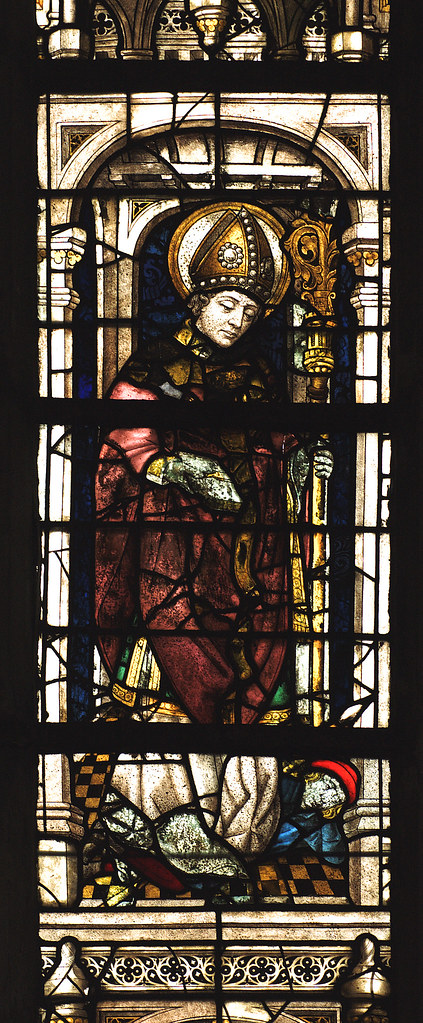The photo captures an intricately detailed stained glass window, likely from a Catholic Church, depicting a solemn religious scene. Dominated by dark hues interspersed with gold and white panels, the tall, narrow window showcases a bishop, discernible by his deep burgundy robe and ornate hat. He holds a golden staff adorned with an elaborate, flowering pattern. The bishop's face and fingers are the only visible parts of his body, and he gazes downward. At his feet lies a smaller figure in blue with a red cap, partially obscured but distinguishable against the checkerboard tile floor of black and gold squares. The window, which spans the height of three standard windows, combines predominantly browns, reds, and golds, with accents of green at the lower end of the bishop's vestments, adding to the rich tapestry of the scene.